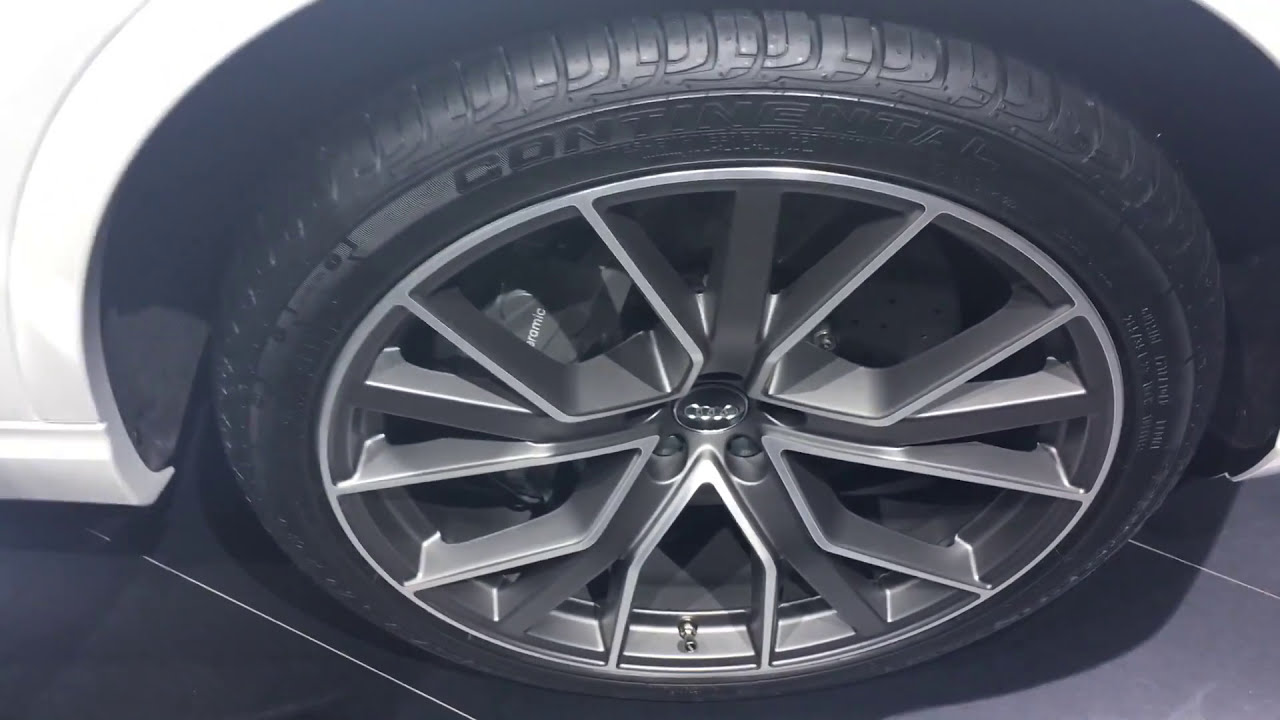This black and white photograph offers an evocative close-up of the wheel well of a white car, likely from Germany. Prominently featured in the image is a detailed view of the vehicle's wheel, equipped with a Continental tire that displays its distinct tread. The wheel sports an Audi logo at its center, surrounded by an intricate mag rim. This rim has a unique design with trapezoidal-shaped spokes that resemble the legs of a spider, each spoke angling upwards before curving down, creating a striking visual effect. Light reflects off these spokes, highlighting their unusual and captivating shape. The dark gray rim, adorned with lighter silver accents, contrasts beautifully with the substantial gray brake calipers visible through the wheel. The photograph captures the interplay of light and shadow, emphasizing the sheen on the top of the tire, although the rest of the branding details on the sidewall remain indistinct. The overall composition of the image, focusing on the intricate and elegant design of the wheel and tire, presents a striking and detailed portrayal of automotive engineering.